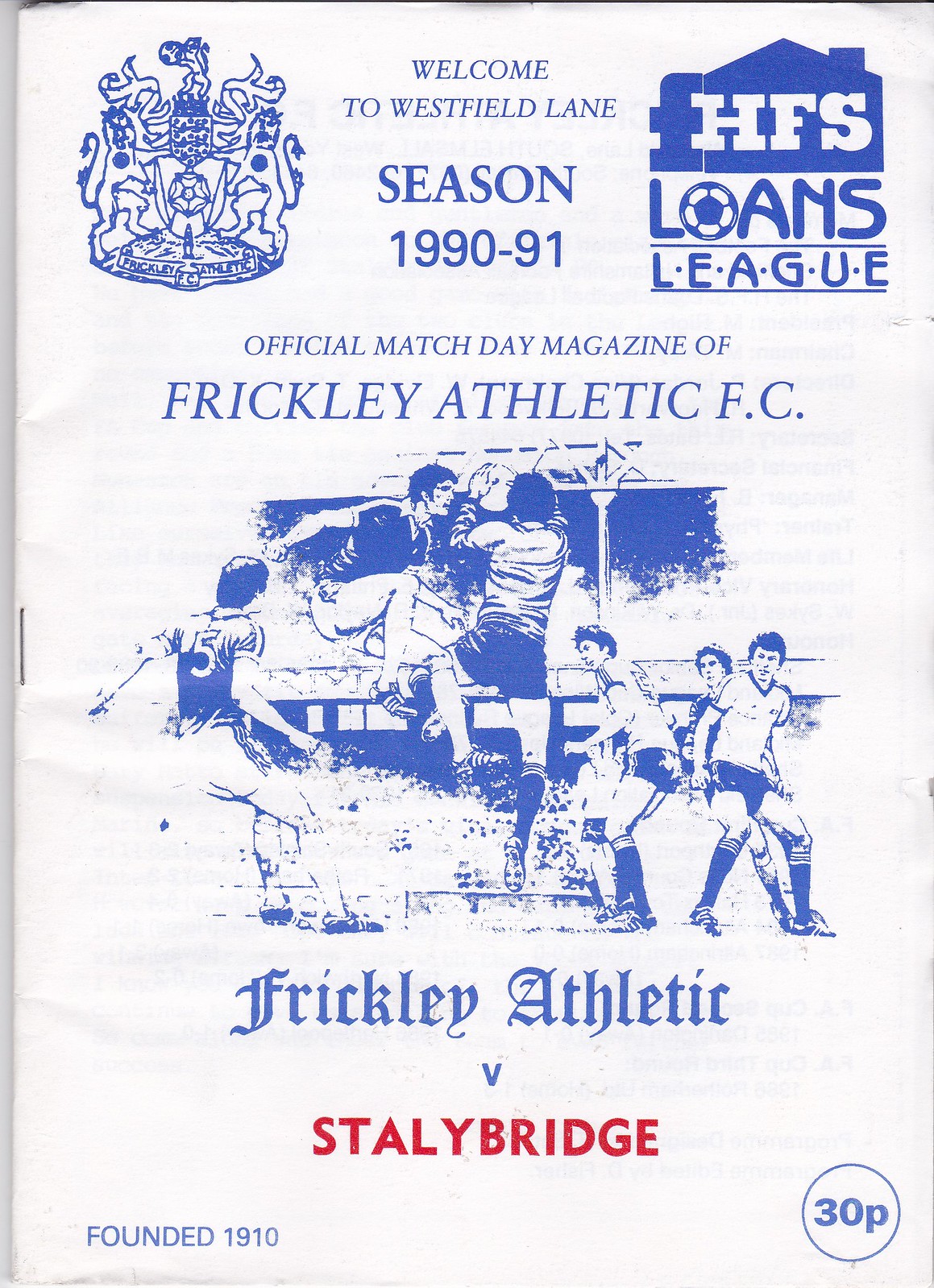This is an official Match Day poster for Frickley Athletic FC's 1990-91 season, prominently titled "Welcome to Westfield Lane." In the top left corner, there's a large emblem, while to its right, the text includes "HFS Loans League," indicating the league name or potential sponsorship. Central to the poster is a bold title that reads, "Frickley Athletic FC," beneath which is a detailed drawing of six men playing soccer in a stadium with seating visible in the background. The match information is clearly highlighted with "Frickley Athletic" in blue followed by a prominent "V" and then "Stolle Bridge" in red. The bottom left corner states, "Founded 1910," marking the club's history, and the bottom right corner indicates the price of "30P" for the program.